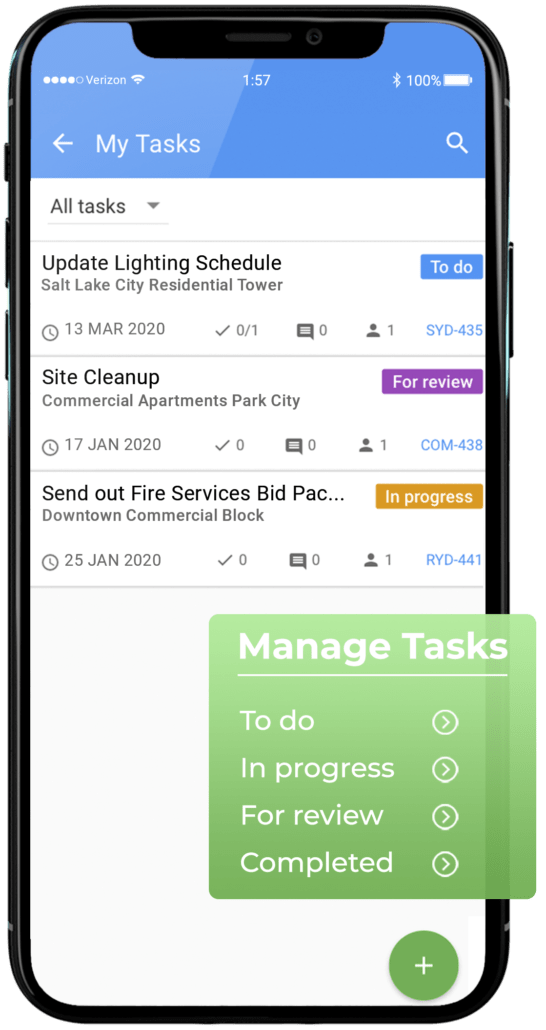The image is a screenshot of a smartphone displaying a task management application. The screen is divided into two main sections: the top half features a gradient of sky blue, baby blue, and darker blue colors. Within this section, four white-highlighted dots are positioned, likely indicating some form of status or progress. Adjacent to these are icons for Verizon signal strength, Wi-Fi, Bluetooth, and a 100% full battery. The time is shown as 1:57 PM. 

To the right of these icons is a search bar. Beneath this colorful header, the screen transitions to a white background where the main content is presented in a vertical list format.

At the top of this list is a dropdown tab labeled "All Tasks." This is followed by a list of tasks displayed in descending order. Each task includes detailed information:

1. **Task: Update Lighting Schedule**
   - **Location:** Salt Lake City Residential Tower
   - **Due Date:** 13 March 2020
   - **Status Icons:** Clock icon (due date), checkmark, comment box with zero comments, and user icon with number one indicating assigned person.
   - **Category:** To-Do
   - **Identifier:** S.Y.D. - 435

2. **Task: Site Cleanup**
   - **Location:** Commercial Apartments, Park City
   - **Due Date:** 17 January 2020
   - **Status Icons:** Clock icon (due date), checkmark, comment box with zero comments, and user icon with number one.
   - **Category:** Full Review
   - **Identifier:** C.M.O. - 438

3. **Task: Send Out Fire Services Bid Pack**
   - **Location:** Downtown Commercial Bank Block
   - **Due Date:** 25 January 2020
   - **Status Icons:** Clock icon (due date), checkmark, comment box with zero comments, and user icon with number one.
   - **Category:** In Progress
   - **Identifier:** R.Y.D. - 411

At the bottom of the screen is a blue and green box containing navigation options for managing tasks, labeled "To Do," "In Progress," "For Review," and "Completed," each with a right-facing arrow. Additionally, there is a green circle with a white plus sign, likely a button to add a new task.